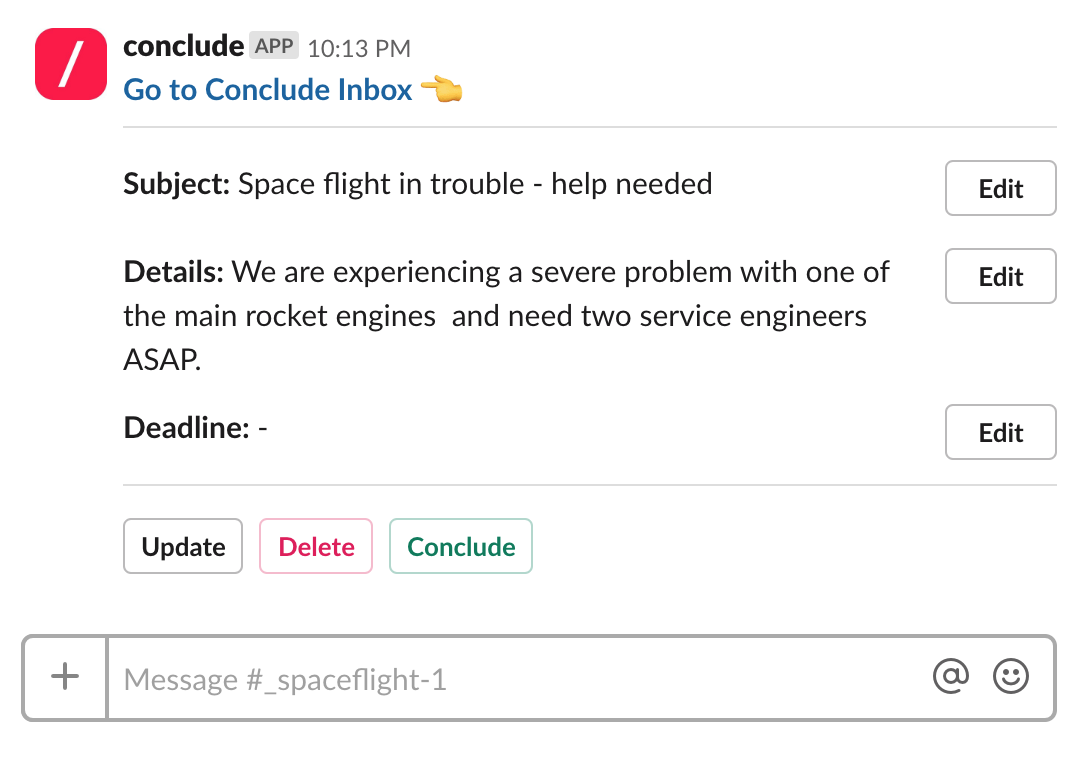The image displays a user interface of an application with several elements. At the top, a red box with a white diagonal line contains the caption "Conclude App 10:13 PM." Below this, blue text reads "Go To Conclude Inbox," accompanied by a yellow index finger icon pointing at it. A light gray horizontal line separates this section from the next. 

Under the line, the text "Subject: Space Flight and Trouble - Help Needed" is displayed. To the right, there are three vertically stacked edit buttons. Following the subject area, there’s a detailed message that reads: "Details: We are experiencing a severe problem with one of the main rocket engines and need two service engineers ASAP." 

Below this, another label reads "Deadline" followed by a light gray line. Underneath, there are boxes labeled "Update" in black, "Delete" in purple, and "Conclude" in dark green. Finally, a text box is located below these options, marked with a plus symbol on the left and containing the text "Message: #_Space Flight-1."